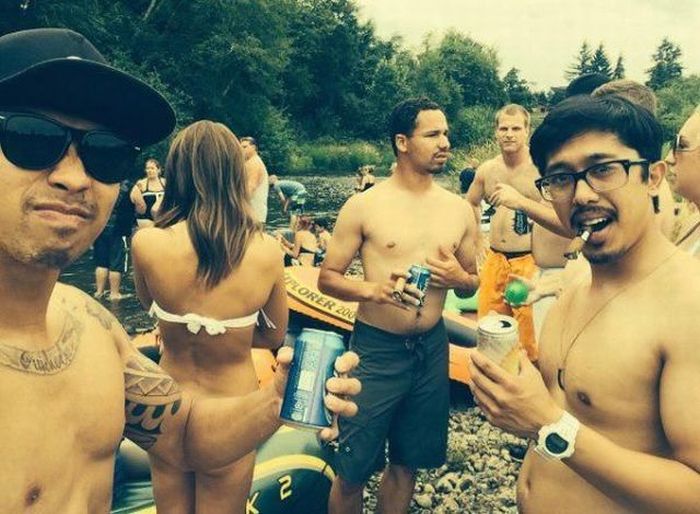In this lively photographic image, a group of people are enjoying a party by a shallow creek. The festive atmosphere is evident as many are holding beers and cigars, basking in the sunny outdoor setting. Two individuals, a man and a woman, are prominently smiling at the camera. The man, wearing glasses and holding a Bud Light, has his arm bent upwards in a peculiar way that creates an amusing optical illusion. It appears as though his arm is the woman's backside, making it look as if she has no bottoms on—an effect that adds a humorous touch to the scene, whether it was intentional or not.

To the left, another man stands out with a cigar clamped between his teeth and glasses perched on his nose. He raises a cheerleader drink or possibly a wine cooler or seltzer, grinning widely for the camera. Behind them, the creek is populated with shirtless men and the occasional person on a blow-up boat, contributing to the overall carefree and casual vibe of the outdoor gathering.